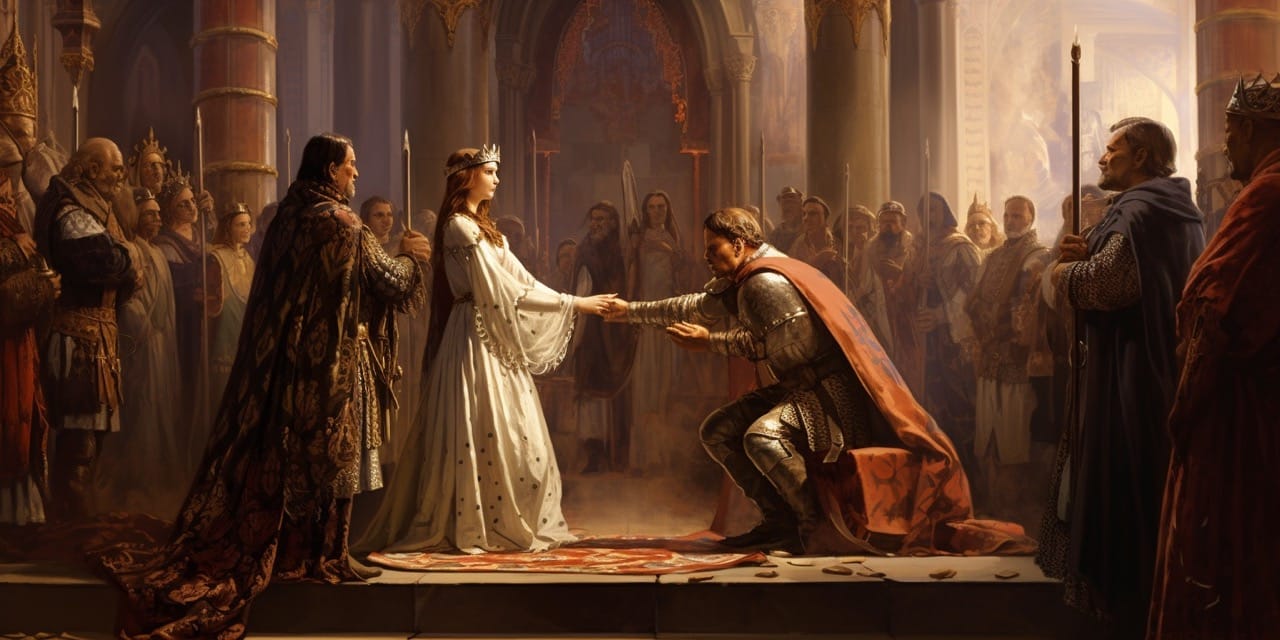This vibrant, full-color painting, likely from the medieval period, captures an indoor scene illuminated by natural light streaming in from the background. The painting, which fills a vertically rectangular canvas, depicts what appears to be a ceremonial or court setting. Central to the composition is a seated man dressed in silver metal armor with a striking long red cape cascading down his back and over the bench he occupies. He is reaching out and holding the hands of a woman standing before him, who is adorned in a long, flowing white dress with large, wide sleeves and a crown on her head. The woman’s auburn hair complements her regal attire. Behind the woman, there is an ornately dressed man, also wearing a long embroidered cape, who appears to play a significant role in the scene. Surrounding these central figures are several individuals, some holding wooden staffs or spears, all under the arches that recede into the background of the hall. The floor features a circular rug, adding a touch of elegance to the setting. The light from outside creates a dramatic illumination, highlighting the main figures and casting shadows that accentuate the depth and grandeur of the hall.